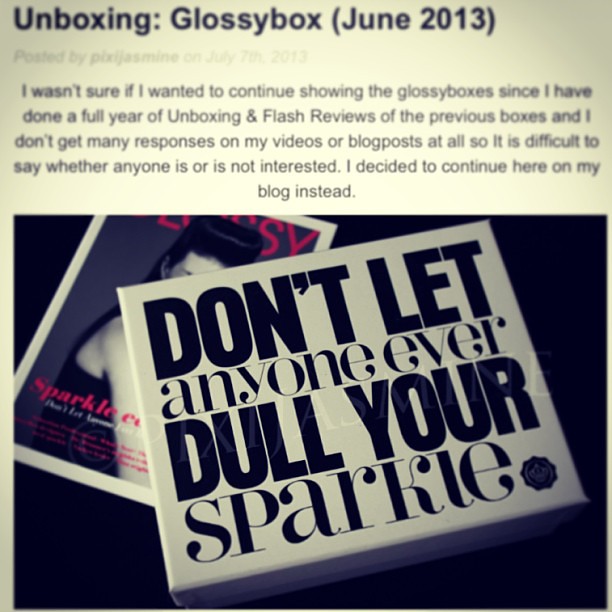The image appears to be a screenshot from a blog post titled "Unboxing: Glossy Box, June 2013." The main focus is on a white box with the phrase "Don't let anyone ever dull your sparkle" written in dark, stylized text. The background shows a slightly blurry cover of a magazine or the top portion of the blog post, featuring an image of a woman partially obscured by the white box. The text of the post reveals the author's contemplation on whether to continue posting glossy box reviews after a year of unboxings and flash reviews, despite the lack of engagement on their previous videos and blog posts. The excerpt reads, "I decided to continue here on my blog instead." The timestamp indicates it was posted by Pixie Jasmine on July 7th, 2013.